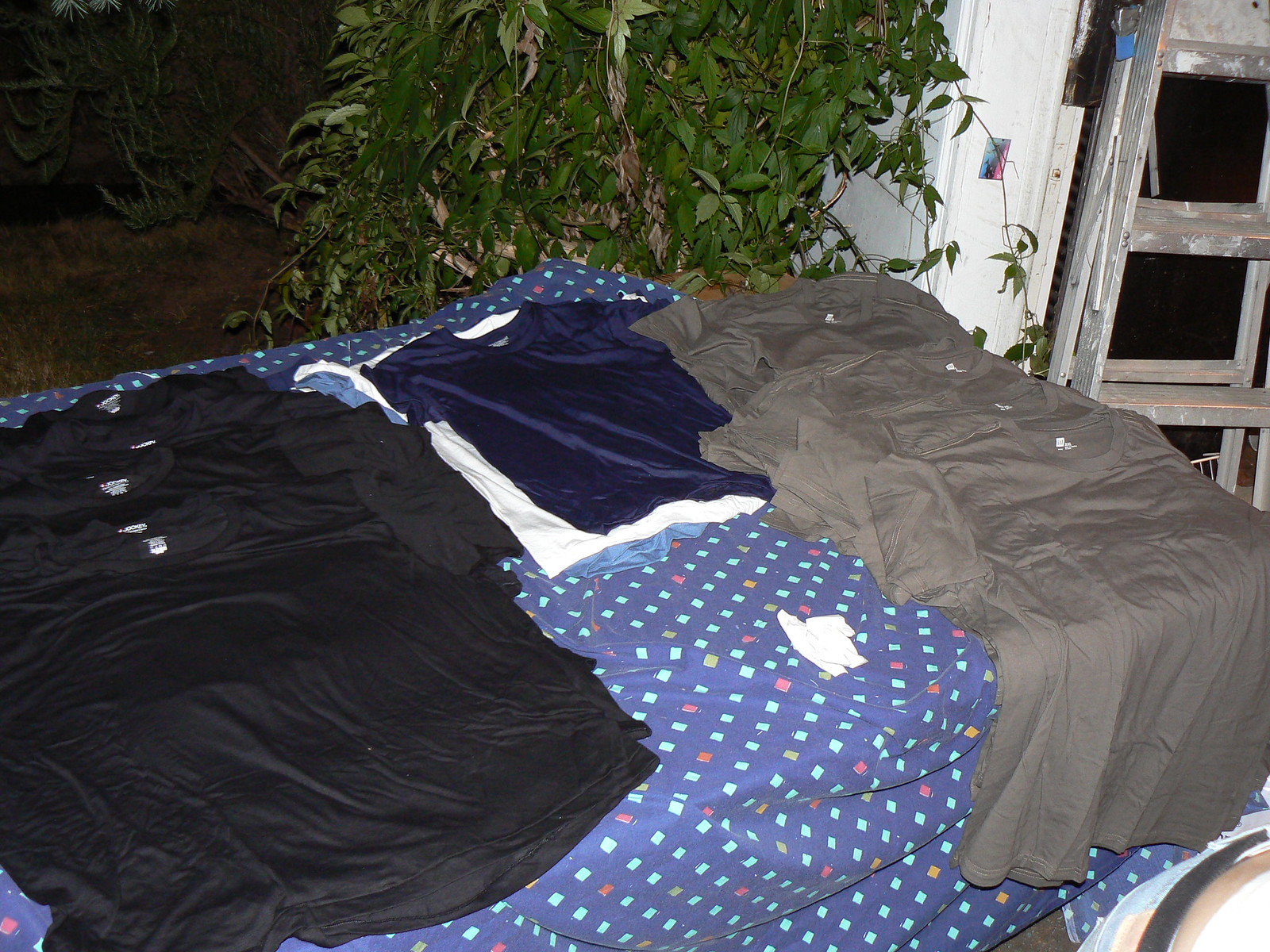The image depicts a nighttime outdoor setting, illuminated by flash, with a mix of natural and artificial elements. The main focus is a twin-size bed or table draped in a medium blue sheet adorned with a pattern of teal blue, reddish, and mustard yellow diamonds. Atop the sheet lies an assortment of shirts. On the left, there are four black Jockey brand shirts, all unfolded and stacked on top of each other. In the center, a navy blue shirt sits on a white shirt, which is beneath a blue shirt. The right side features about five dark gray Gap shirts. Surrounding this setup, leaves and trees are visible in the background, suggesting an outdoor environment, while a white wooden door frame and a light grey folding metal ladder appear on the right-hand side, indicating proximity to an indoor area. A green bush rises beside the door frame, adding to the natural surroundings.